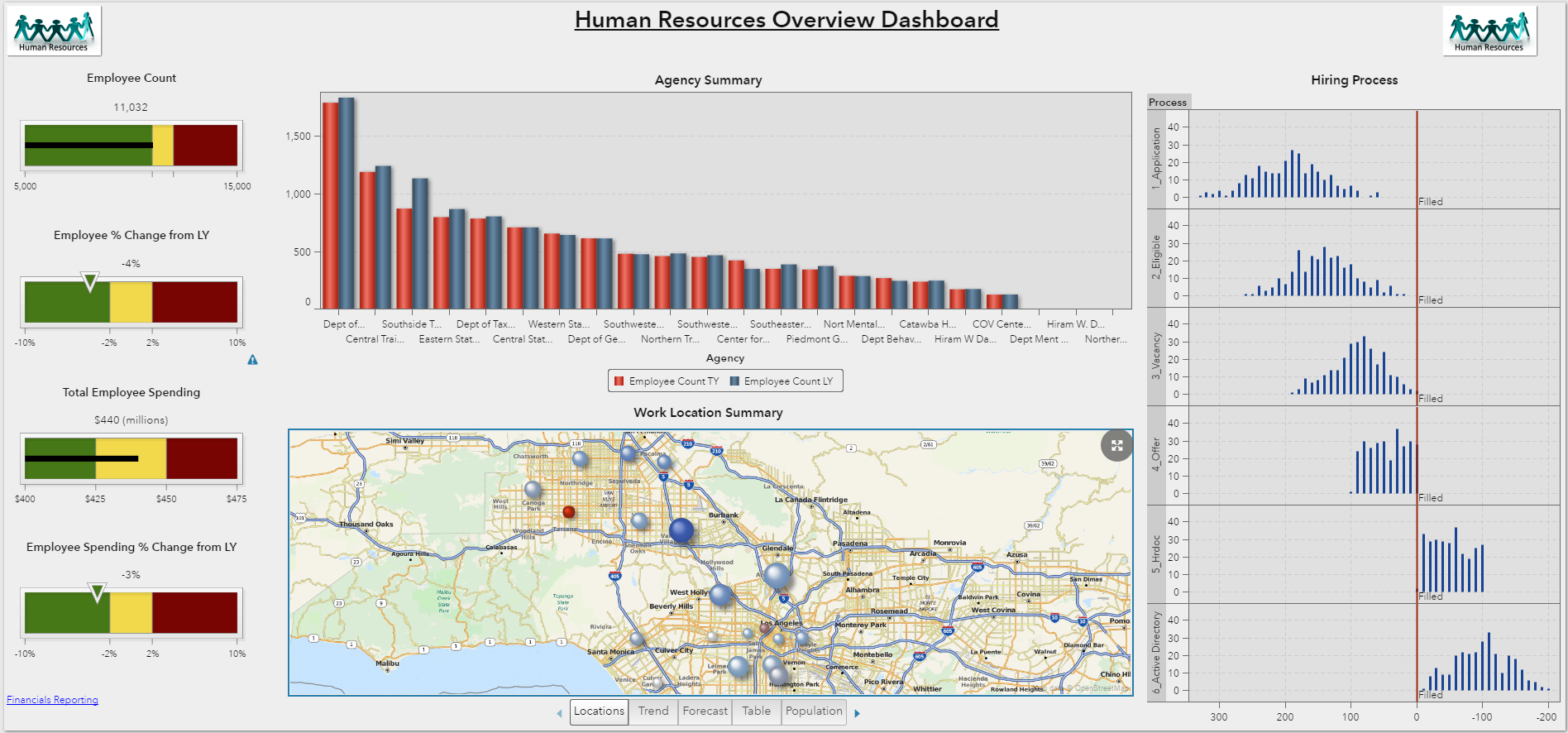This digital information image, set against a light gray background, is titled "Human Resource Overview Dashboard" in black text at the top center. Just below, "Agency Summary" appears in smaller black font. The top corners feature logos that read "Human Resource" with green or bluish characters. 

Central to the image is a vertical line graph, showcasing department names along the x-axis and numerical values (0, 500, 1000, 1500) on the y-axis. This graph uses red and blue lines to convey employee count across various departments like the Department of Tax and others.

Below the graph is a state map, predominantly cream-colored, interlaced with blue and yellow lines resembling highways. The map is dotted with blue circles at various points and a solitary red circle, adding layer of spatial data visualization.

On the left side of the image, four rectangular boxes represent statistics using varying amounts of green, yellow, and red colors. These color segments detail different data points or progress metrics.

To the right, a series of additional graphs, characterized by dark blue vertical lines, possibly represent various stages or stats of the hiring process, adding more depth to the overall dashboard.

The dashboard provides a holistic overview with clear visual representations through multiple charts, maps, and statistics, aiding comprehensive human resource analysis.